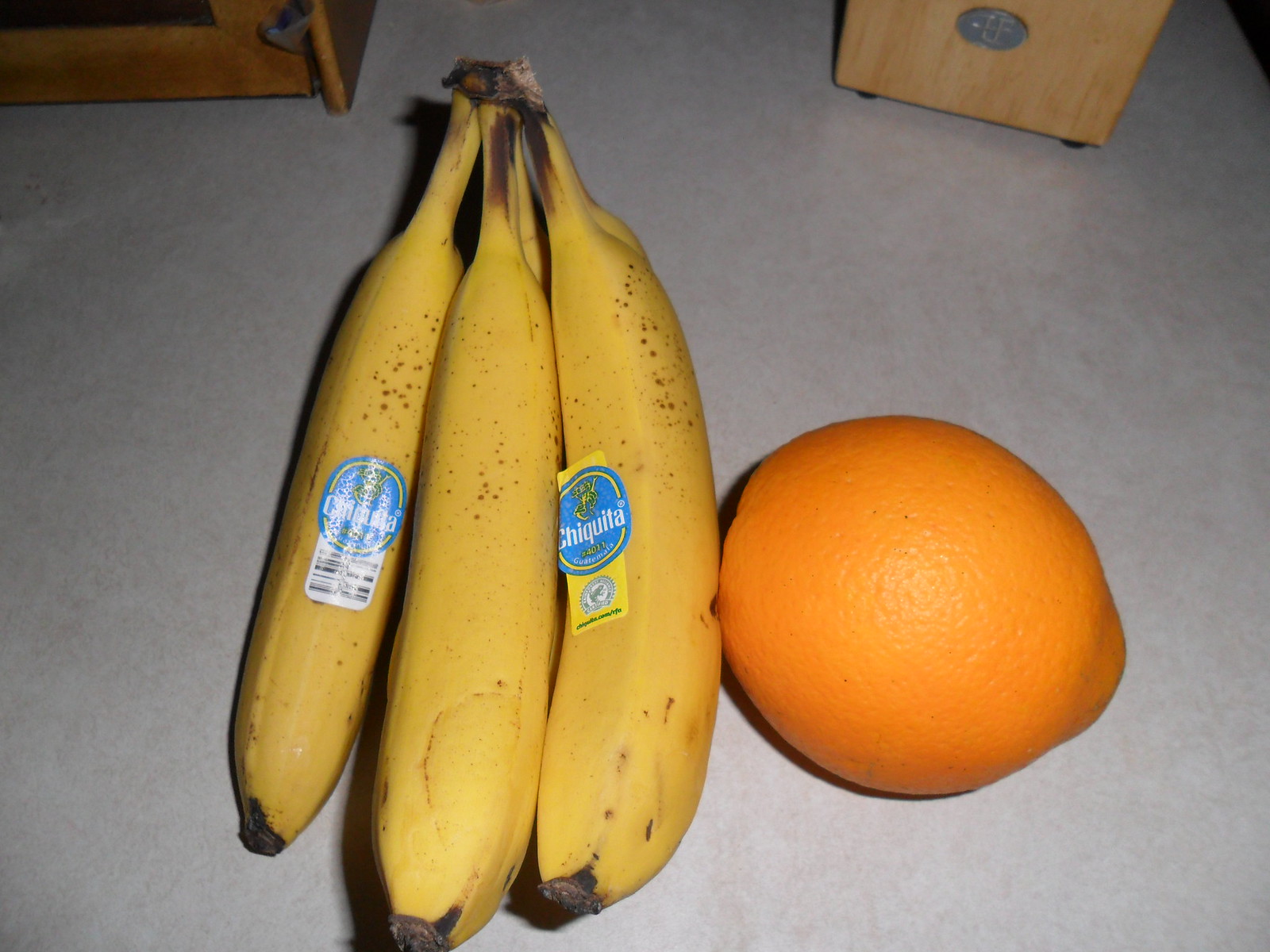In this top-down view of a white table, five bananas are neatly arranged on the left side, four of them bearing the distinctive blue Chiquita emblem, with the left-most banana also featuring a white-and-black barcode sticker. An orange rests independently on the right side of the table. The background offers added texture with a partially visible brown wooden box in the top left corner, and a second wooden box on the right side, adorned with a silver emblem. The entire scene is set indoors, potentially in a shop, providing a clean and organized display of fresh fruit.